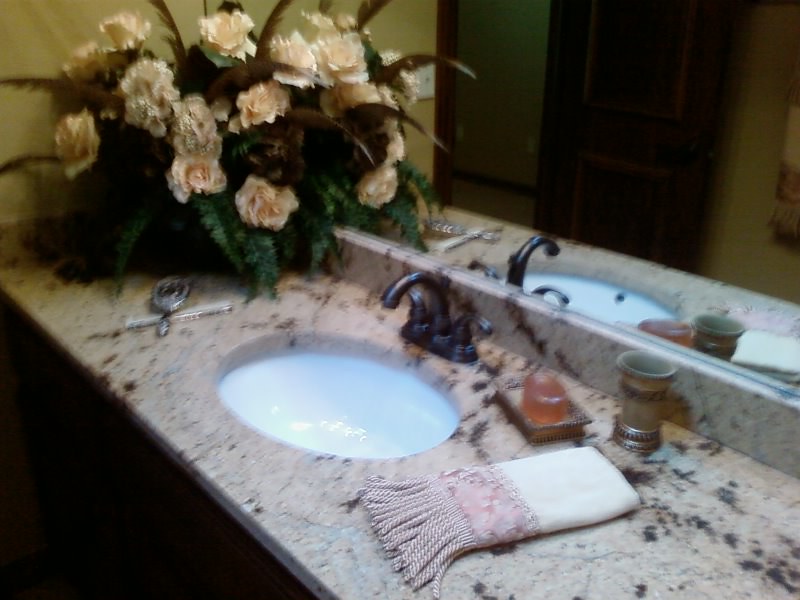The image depicts a sophisticated, high-end bathroom interior. The countertop, made of a luxurious beige marble adorned with black and white speckles, serves as the central feature. A dark bronze faucet with dual handles complements the pristine white basin, reflecting an elegant design. To the right, a neatly folded beige towel with tassels adds a touch of softness, while beside it sits a distinguished bronze cup embellished with intricate designs.

To the left of the sink, an orange bar of soap rests in a bronze tray, exuding a warm, inviting vibe. Adjacent to it stands a grand bouquet, its beige flowers intertwined with brownish foliage and green leaves, infusing the space with natural charm. Below the bouquet, a silver hairbrush and comb lie in wait.

The mirror above the sink captures the reflection of a brown door and its frame, alongside a wall where a small towel is neatly hung. The lower part of the image reveals a darkened area beneath the countertop, completing this elegantly composed bathroom scene.